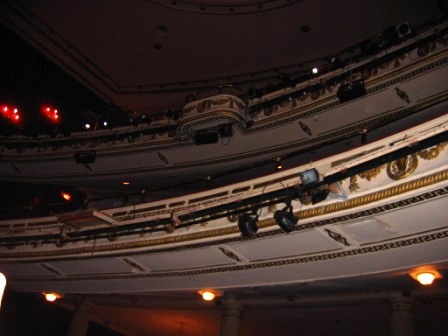This image captures the grand interior of an opulent theater or auditorium from the perspective of someone standing on the ground floor, looking up towards two levels of balconies. The balconies are predominantly white with ornate gold trims that accentuate their elegance. Each level features house lights along the bottom edges, with additional red lights likely serving as exit signs or emergency indicators. The middle balcony has spotlights hanging down, presumably to illuminate the stage or assist with visibility in the auditorium. The top level contains black boxes that might be speakers. The ceiling is a mix of white and dark brown hues, possibly due to the lighting conditions or shadows. The entire space is intricately designed, with pillars on the ground level supporting the upper tiers, creating a grand and sophisticated atmosphere reminiscent of a ballroom or operatic theater. The flash of the camera enhances the illumination of the balconies against the high, dark ceiling, further emphasizing the theater's majestic architectural details.